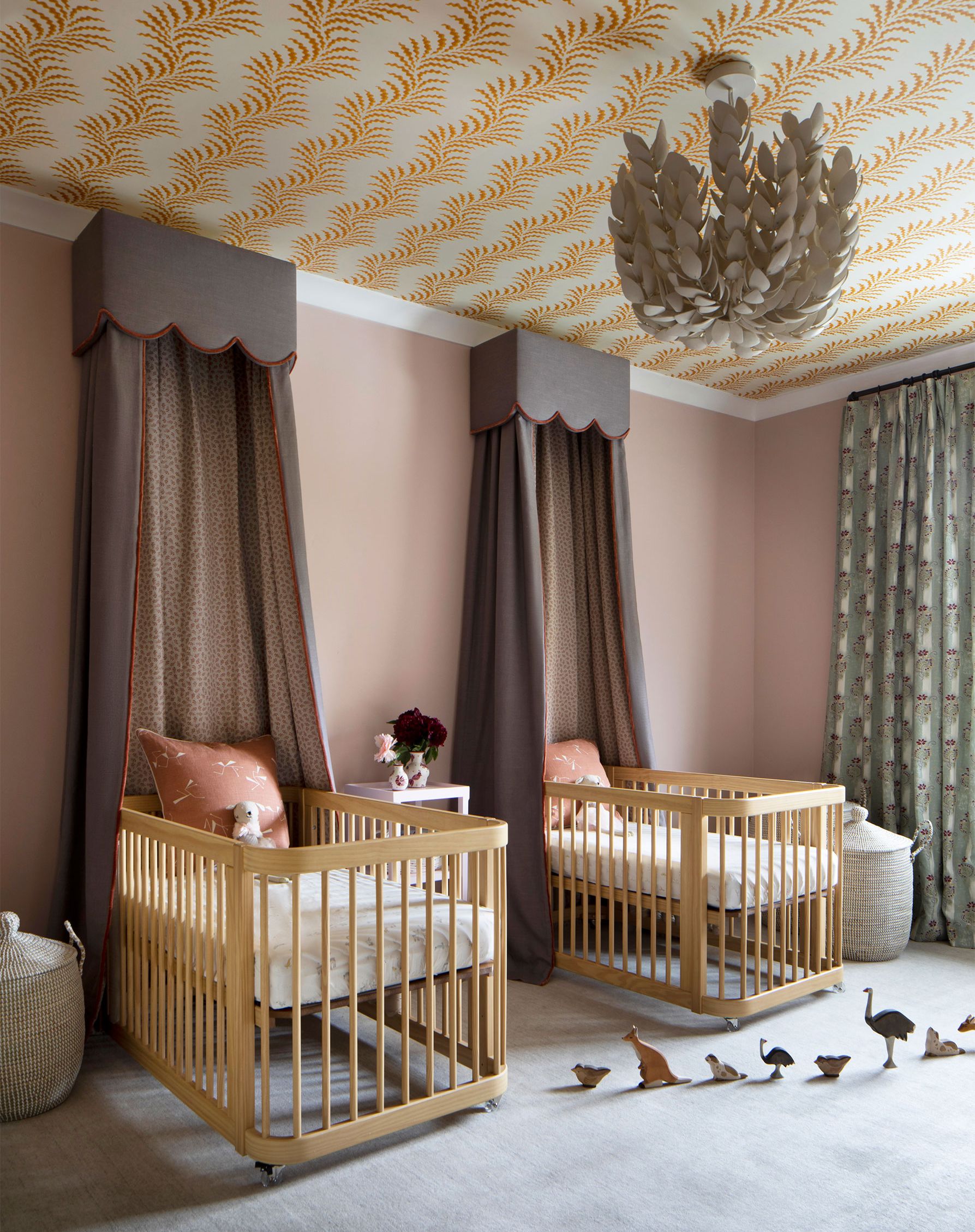This color photograph showcases an elegant and high-end baby nursery, detailed with luxurious touches. The room, characterized by its taupe walls and gray carpeted floor, features two light wooden baby cribs situated in a corner. Each crib is adorned with white sheets, a small mattress, purple or pink pillows, and stuffed bears resting against the pillows. Behind the cribs, brown drapes descend from the ceiling, creating a canopy effect. Above the cribs hangs an ornate chandelier-like lamp crafted from grayish white leaves.

The ceiling is decorated with a repeating yellow and white plant design. On either side of the cribs, gray cloth baskets stand, possibly for laundry or diaper storage. In between the cribs is a white side table. The room also includes gray curtains with a subtle polka dot pattern.

Scattered across the gray carpet in front of the cribs are small wooden block toys shaped like various animals, including ostriches, kangaroos, birds, and possibly seals. These toys form a playful pathway leading up to the crib on the left. The meticulous detailing and coordinated color palette emphasize the nursery's sophisticated and inviting atmosphere.